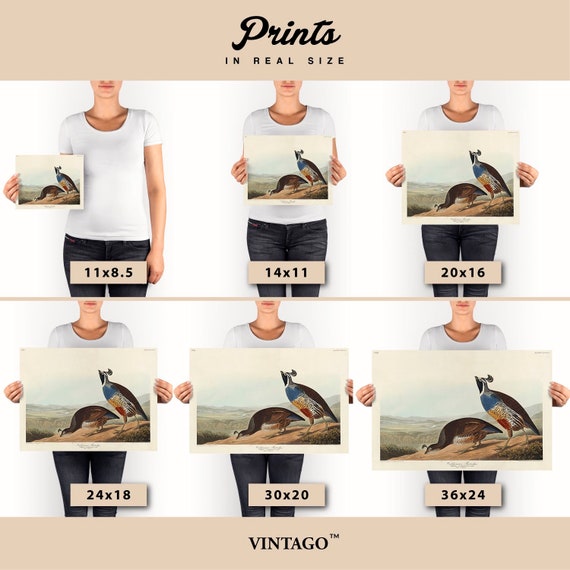The image is an infographic showcasing different print sizes compared to a person's body for visual reference. It features a woman standing in two rows, with three versions of herself on the top row and three on the bottom row, all holding prints of the same image of two pigeon-like birds in a landscape. The woman's face is partially visible from the bottom of her nose to her mouth, and she is wearing a white short-sleeved shirt and dark blue denim jeans.

At the top of the image, the text reads "Prints in Real Size" and the bottom features the brand name "Vintago." Each position shows her holding a larger print size starting with an 11x8.5 inch print held in one hand. Sequentially, she holds a 14x11 inch print, a 20x16 inch print, a 24x18 inch print, a 30x20 inch print, and finally a 36x24 inch print, all in two hands. The smallest print, 11x8.5 inches, appears diminutive compared to her body, while the largest, 36x24 inches, is nearly twice her width, providing a clear and comparative visual scale of the print sizes.